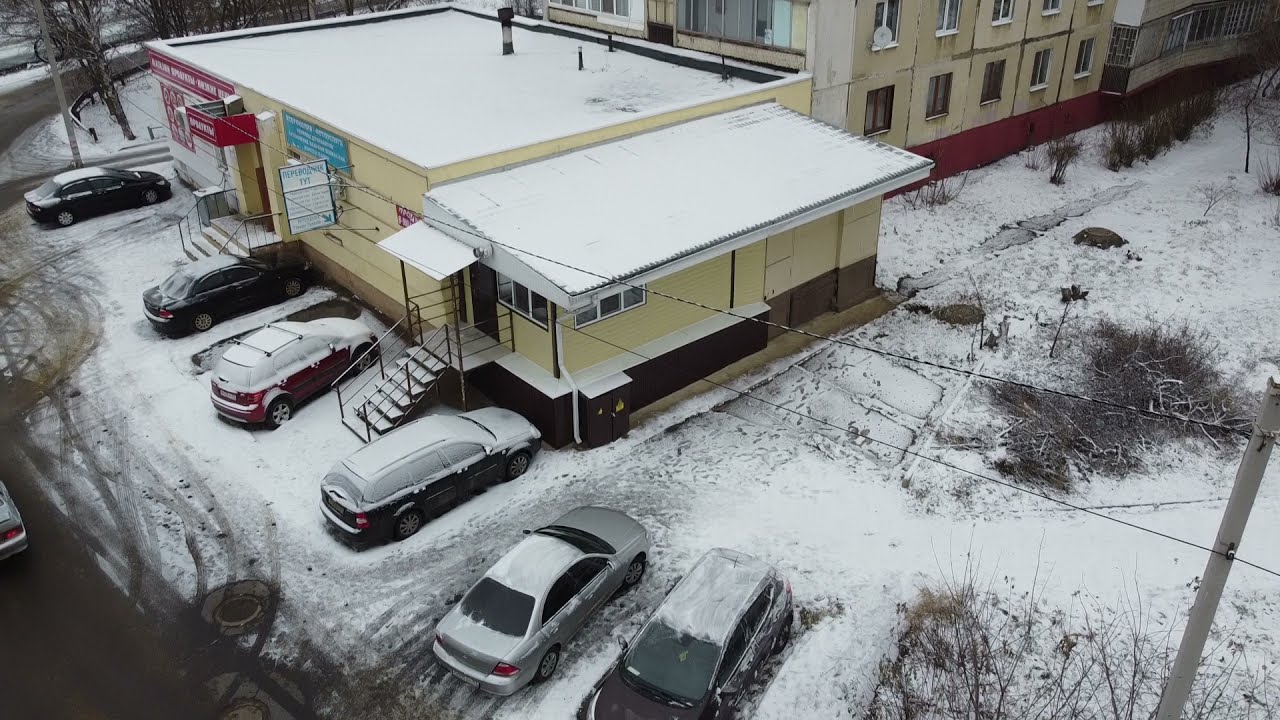On a snowy winter day, this outdoor photo captures an overhead view of a parking lot adjacent to a small, one-story yellow building with a flat rooftop and a white awning extending from its eaves. The lot features six parked cars, partially covered in slushy, melting snow. In the lower left corner, a dark gray, wet street is visible with moving cars. To the right of the street, the row of parked cars, including a mix of small cars and SUVs, stretches along the building, which has two sets of stairs leading to its entrances. The building sports red and blue signage, the details of which are unclear. In the background, a taller, two-story building with a red-brick bottom and off-white upper floors provides contrast. The lower right corner includes snow-covered fields with dead brush and visible power lines. The overall scene is a testament to the cold, snowy weather enveloping this urban area.